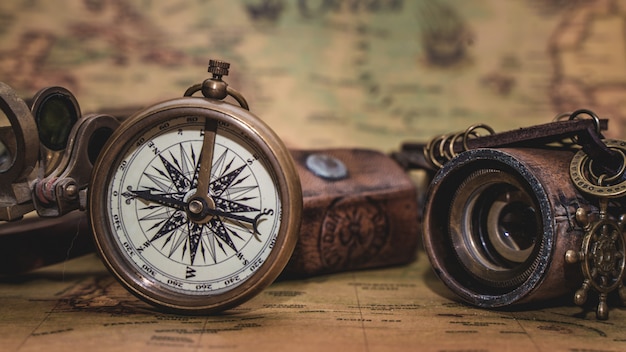The image is a detailed close-up photograph of various decorative exploration tools elegantly arranged on a blurred Old World styled map, mostly on beige parchment, detailed with unreadable black text and splotches of greens, browns, and blacks. The centerpiece is an extremely clean compass with a bronze frame and a white face featuring black pointy designs and bold letters indicating the directions W, S, E, with a brown needle pointing upwards. To the right of the compass lies a ship's steering wheel pendant hanging off a vintage-styled spyglass or telescope. The telescope, wrapped in aged-looking brown leather adorned with painted black spots and a black rim, gives it a distinct antique appearance. On the left, a bronze magnifying device with small sliders of glass, purportedly for image enlargement, adds to the Old World aesthetic. Behind the compass rests an indiscernible leather item with a stamped design and a metal snap, partially obscured by the tools in the foreground. The map itself, serving as both the background and base, enhances the historical feel of the scene, effectively showcasing the array of intricate exploration instruments.